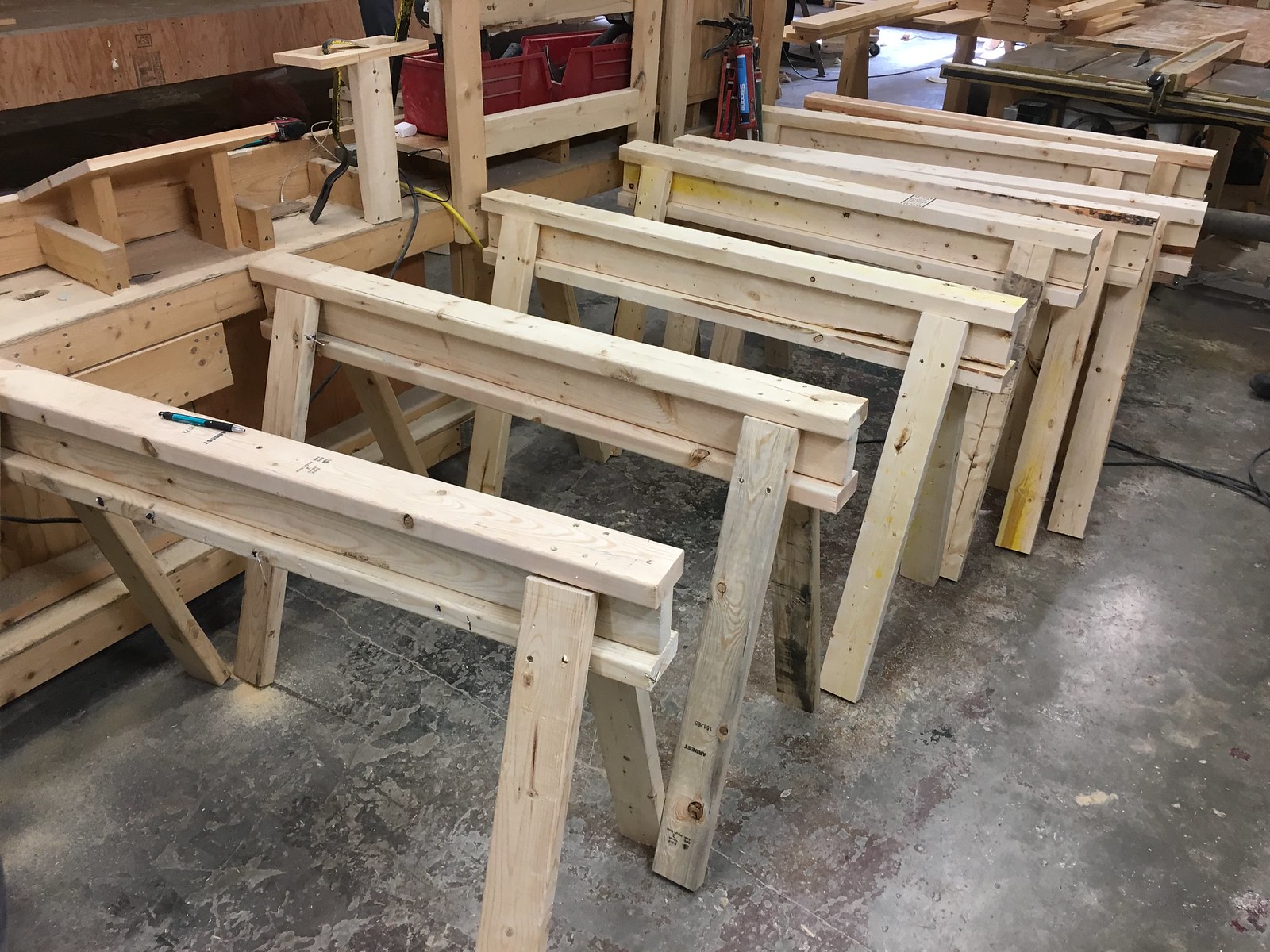This detailed photograph captures a well-lit woodshop, possibly part of a woodshop class or a construction warehouse, with a black concrete floor and various wooden structures in progress. Central to the image are several wooden saw horses lined up in a row. Each saw horse is composed of two slanted two by fours forming triangular legs, a base two by four, a vertical support, and another flat two by four on top. One of the saw horses shows pencil markings, indicating active use. Surrounding these are multiple other wooden projects, shelves, and tools, including a table saw, hinting at an environment where masons and carpenters are at work. Predominantly, the scene features shades of brown with some red accents, highlighting the natural wooden materials being used.